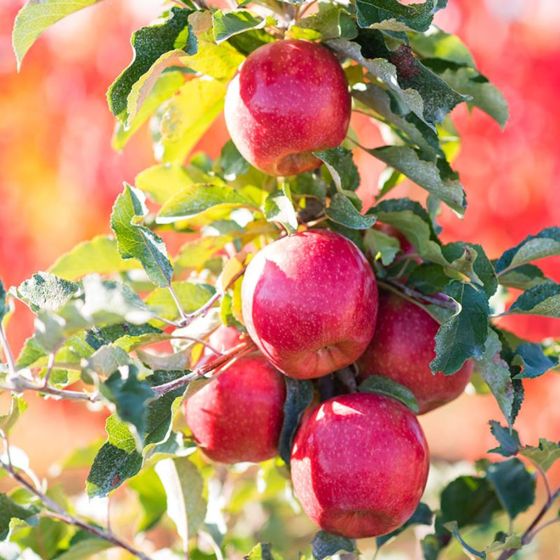In this vibrant outdoor photograph, we see a cluster of shiny, ripe red apples, hanging gracefully from a tree branch. Centered in the image are five prominently featured apples, their glossy skins adorned with tiny spots—a sign of their readiness for harvest. The apples are suspended on delicate light brown twigs, surrounded by a mix of verdant green leaves. These leaves exhibit a beautiful gradient, ranging from pale green where sunlight touches them to a darker green in the shaded areas. 

The sunlight, streaming in from the left, not only highlights the apples but also casts a gentle glow on selected leaves, giving them a yellowish tint. The scene is set against a blurred backdrop of subdued red and pink hues, suggesting an orchard in full bloom. The square photograph, approximately four inches on each side, captures the essence of a bright, sunny day with the garden elements fading softly into the background, allowing the apples to be the focal point of this picturesque moment.